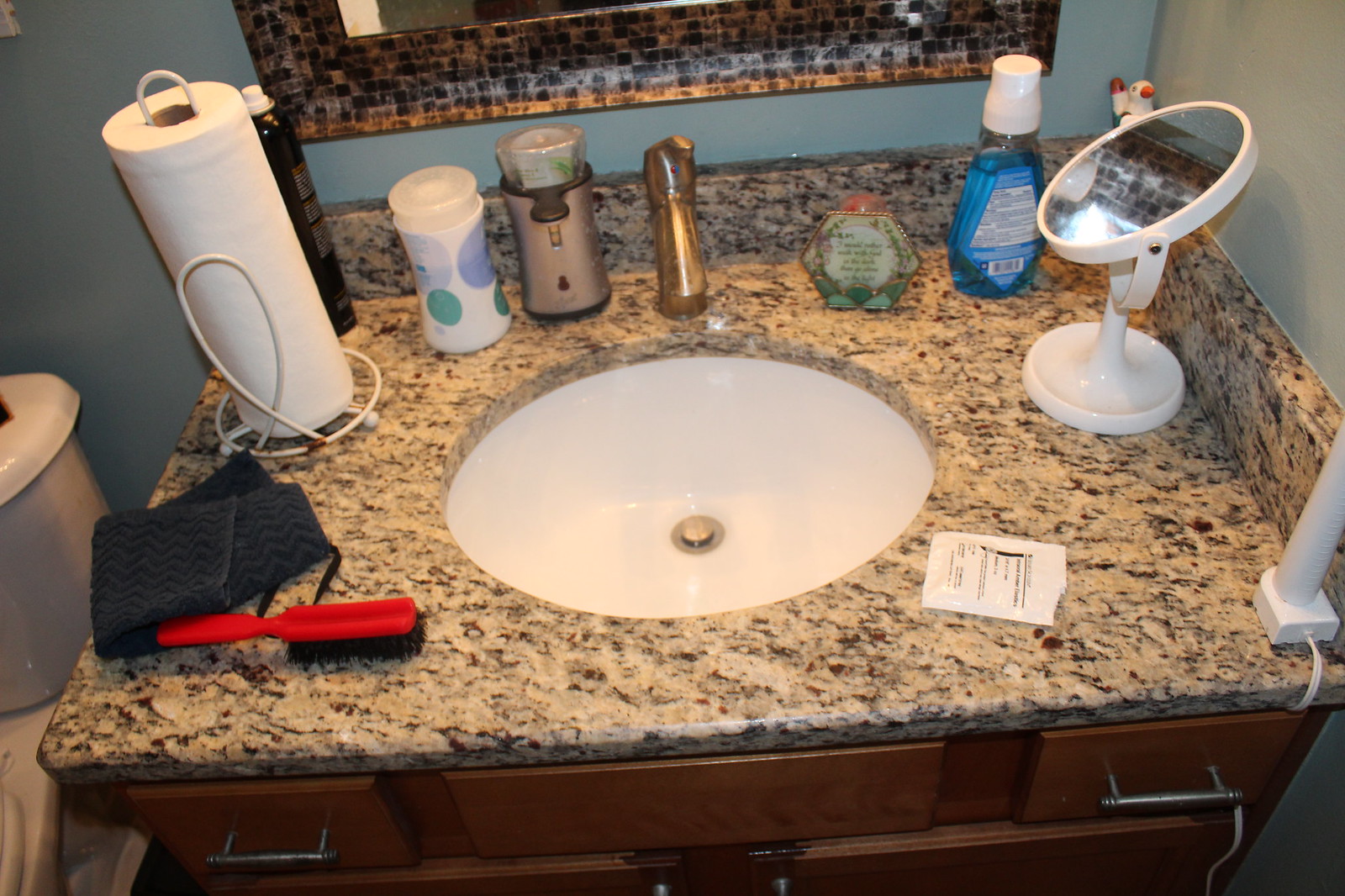The image features a well-appointed bathroom characterized by its detailed elements. On the far left, just barely in frame, is a toilet. The focal point of the photo is the bathroom vanity, which is topped with a speckled white granite countertop interspersed with black, brown, and gray flecks. Centered above the vanity is a mirror bordered with a metallic frame that adds a touch of elegance to the space.

The vanity surface is dotted with various items. A red hairbrush lies prominently on the counter, next to what appears to be the packaging of disposable wipes, suggesting recent use. A roll of paper towels and a neatly folded small towel are also present. An adjustable circular mirror stands on the vanity, offering versatility for different viewing angles. The countertop is further populated with a bottle of mouthwash, a soap dispenser with a stainless steel pump, a canister of hairspray in a black bottle, and another unidentified bottle.

A device, likely an electric toothbrush, is plugged into the wall with its cord trailing down to the counter. The vanity itself is supported by brown wooden drawers, accented with sleek steel handles, adding both functionality and aesthetic appeal to the bathroom setup.